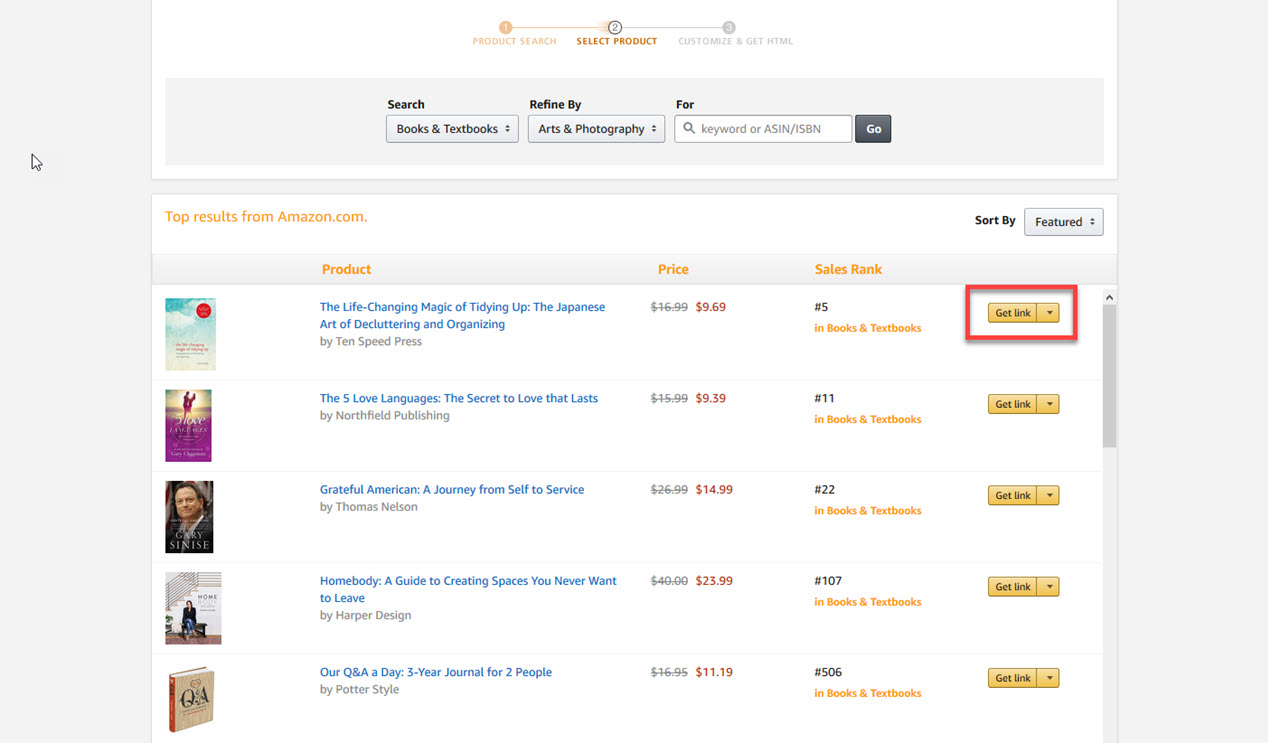The image depicts an online book purchasing interface, likely from Amazon. At the top center of the image, there are three prominent sections. The first section features an orange circle with a white number "1" inside it, labeled "Product Search" below. To its right, the second section has a white background with a black number "2," labeled "Select Product." The third section presents a black background with a white number "3," labeled "Customize and Gift HTML."

Below these sections, there is another row of three categories. The first category is labeled "Search," the second "Refine By," and the third "For." Under the third category is a rectangular text entry field with the placeholder text "Keyword or ASIN/ISBN." Adjacent to this field is a small square button labeled "Go."

The lower half of the image showcases five books available for purchase. The books are arranged in a list with their prices displayed as follows from top to bottom: $9.69, $9.39, $14.99, $23.99, and $11.19.